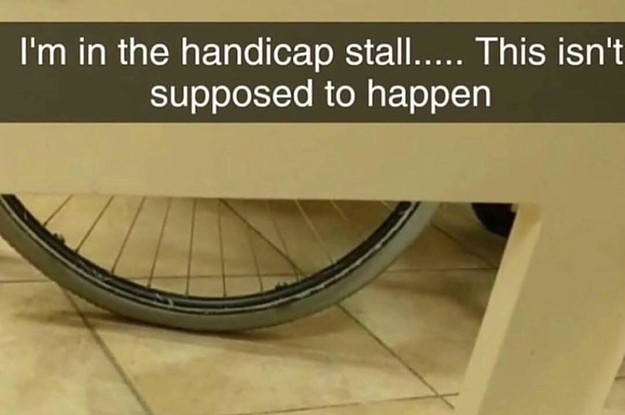The rectangular image features a bathroom stall, with a caption running across the top saying, "I'm in the handicap stall.... This isn't supposed to happen." The caption is displayed in white text on a neutral khaki-colored banner. The stall and surrounding room are in beige tones, including the tile floor. The bottom portion of the stall has a cutout through which a large gray wheelchair wheel, with slightly dirty spokes, is visible. On the right side, either a smaller wheel or a black shoe is partially visible. The image invokes a sense of surprise or an unsettling occurrence within the handicapped stall, although no person can be seen.